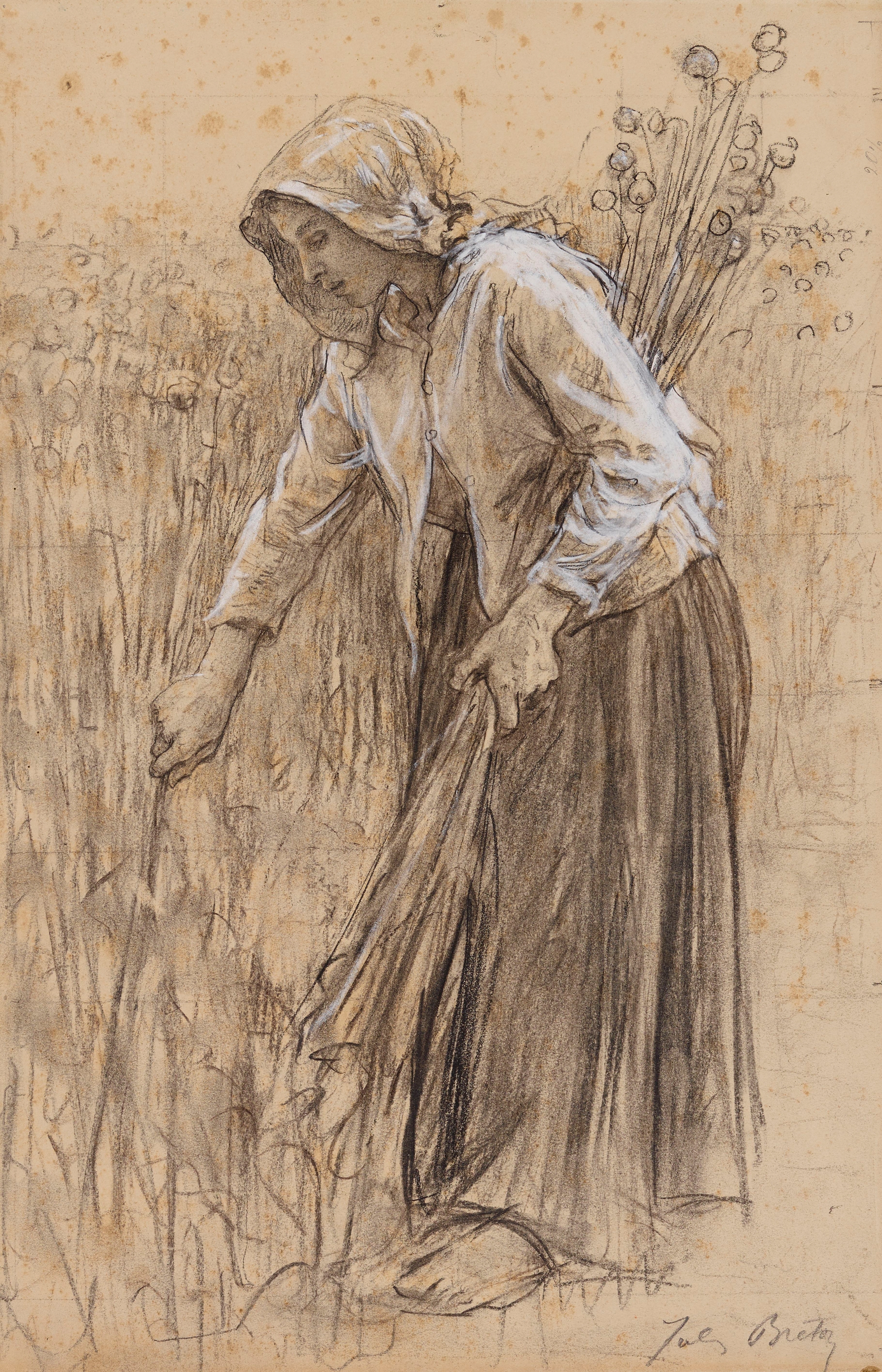In this detailed sketch, rendered in shades of gray, brown, and white on tan paper, we see a barefoot woman standing in an extensive field, possibly of wildflowers or long-stemmed wheat. She is dressed in a dark, flowing skirt that reaches down to her feet, a white blouse, and a white headscarf or headdress tied around her head. The woman, captured in profile facing left, has an armful of incredibly tall plants — almost reaching her shoulders — cradled in her left hand while she reaches down with her right hand to pull another stalk from the ground. The scene conveys a rhythmic, labor-intensive action in a lush, expansive field. The tall plants, indistinguishable in type due to the monochromatic medium, dominate the background, adding depth to the rustic setting. The bottom right corner features a signature, possibly starting with a "Z" and a "B," hinting at the artist's identity. This pencil drawing, highlighted with some white accents, profoundly captures the essence of rural life and meticulous handcraft.